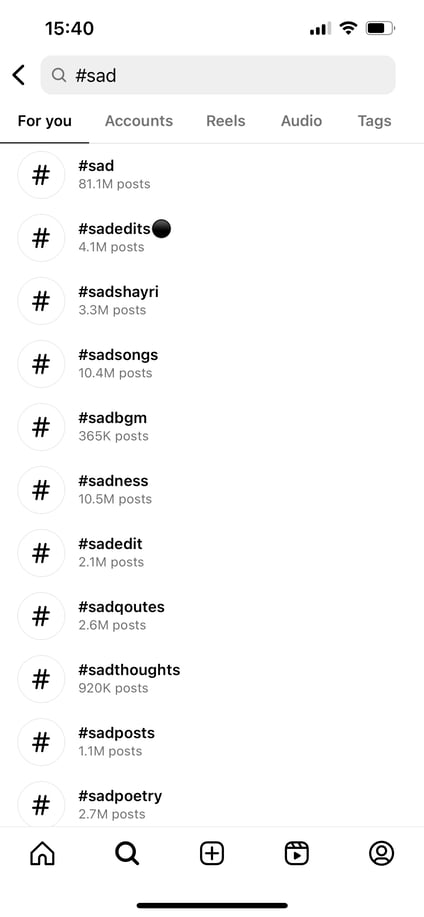The image depicts the results of a search on a mobile phone. The screen shows a search query for the hashtag "sad" at 15:40, under the heading "For You." The search results consist of a list of entries starting with various "sad" related terms: #sad, #sad edits, #sad shire, #sad shiree, #sad songs, #sad BGM, #sadness, #sad edit, #sad quotes (this appears to be a peculiar-looking 'Q' and not a misspelling), #sad thoughts, #sad posts, and #sad poetry. A black dot is positioned beside "#sad edits," suggesting it may be selected, potentially leading to a page full of 'sad edits.' Overall, the screen has a somewhat melancholic appearance.